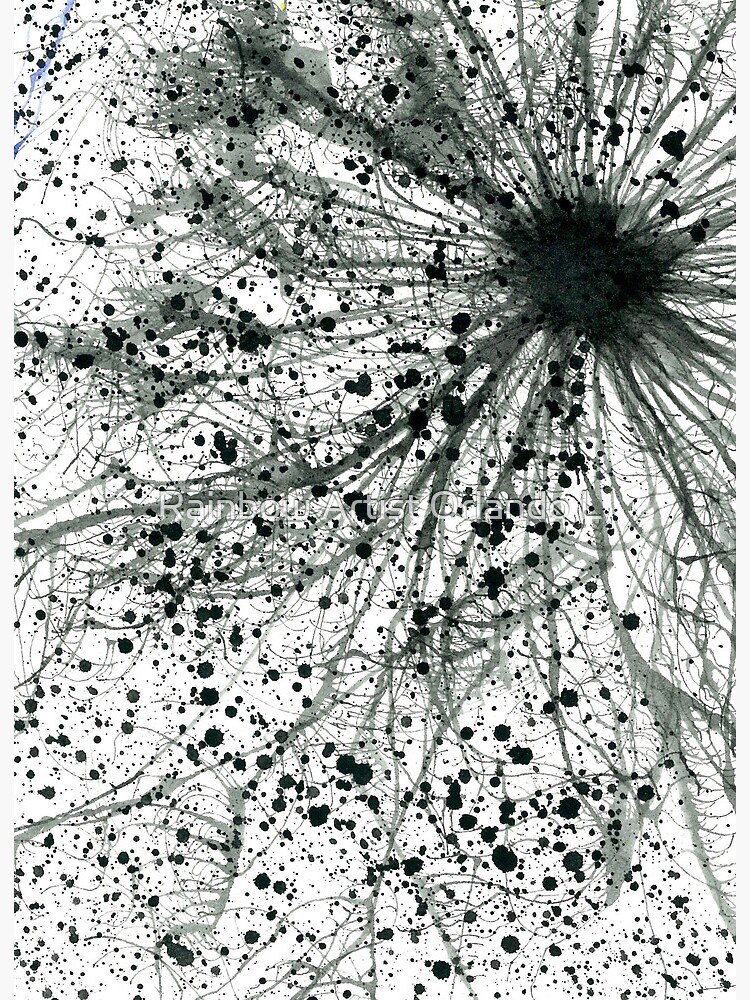A vertically rectangular black and white image, possibly modern art, with a white background. Dominating the upper right corner is a black, cell-like sphere from which numerous thin, gray, tentacle-like fibers radiate outward, resembling an intricate web spreading across the entire piece. These fibers branch out extensively, creating a complex network. Scattered throughout the image are dozens of black splotches, similar to paint or ink spots. In the center of the image, a faint watermark reads "rainbow artist Orlando" in almost transparent white text with gray shading.